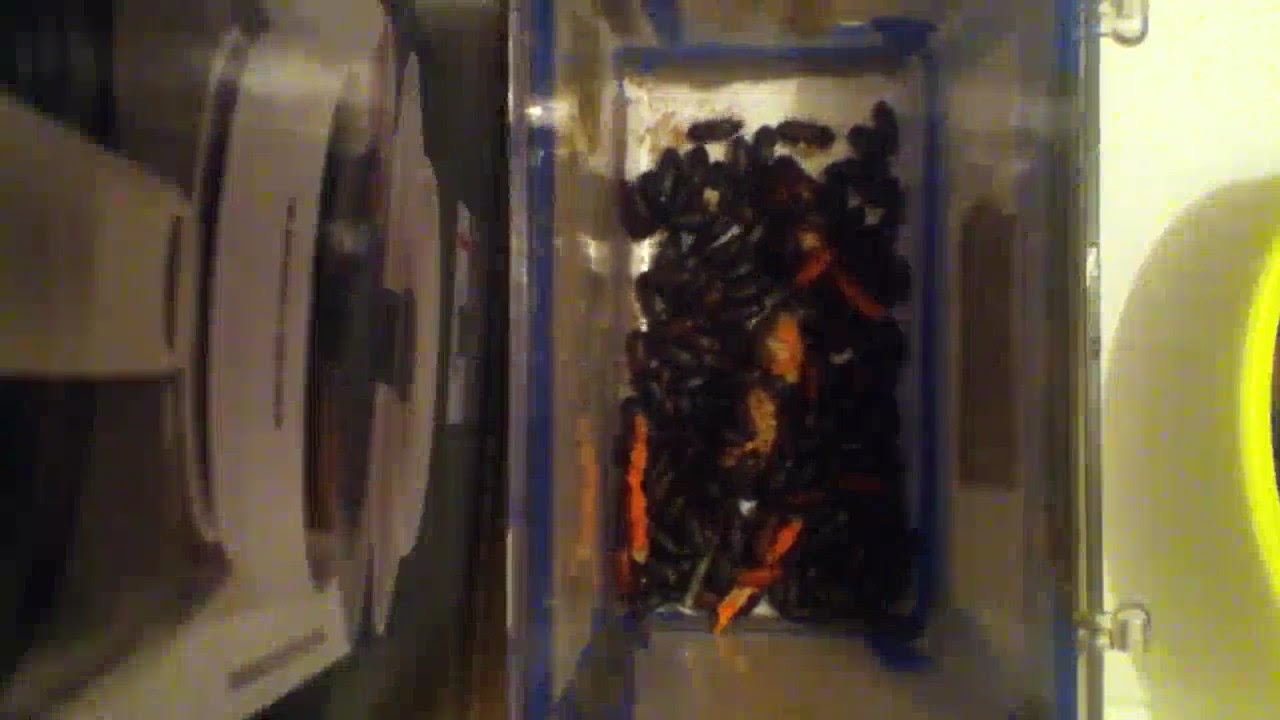The image features a somewhat blurry, horizontal still from a video, centered on a tall rectangular plastic container filled with countless small, black ovoid shapes, resembling bugs or cockroaches. The container's bottom is cluttered with what appears to be waste and several orange items, possibly food for the bugs. Blue highlights adorn the container, with markings around its upper and lower edges, and plastic hinges suggesting it might have a lid. To the left of the container stands a gray appliance with a large circular feature, potentially a washing machine or dryer. On the right side, the setting transitions to a flat, white surface resembling a floor, with a yellow tub nearby, adding to the indeterminate but cluttered environment of the scene.